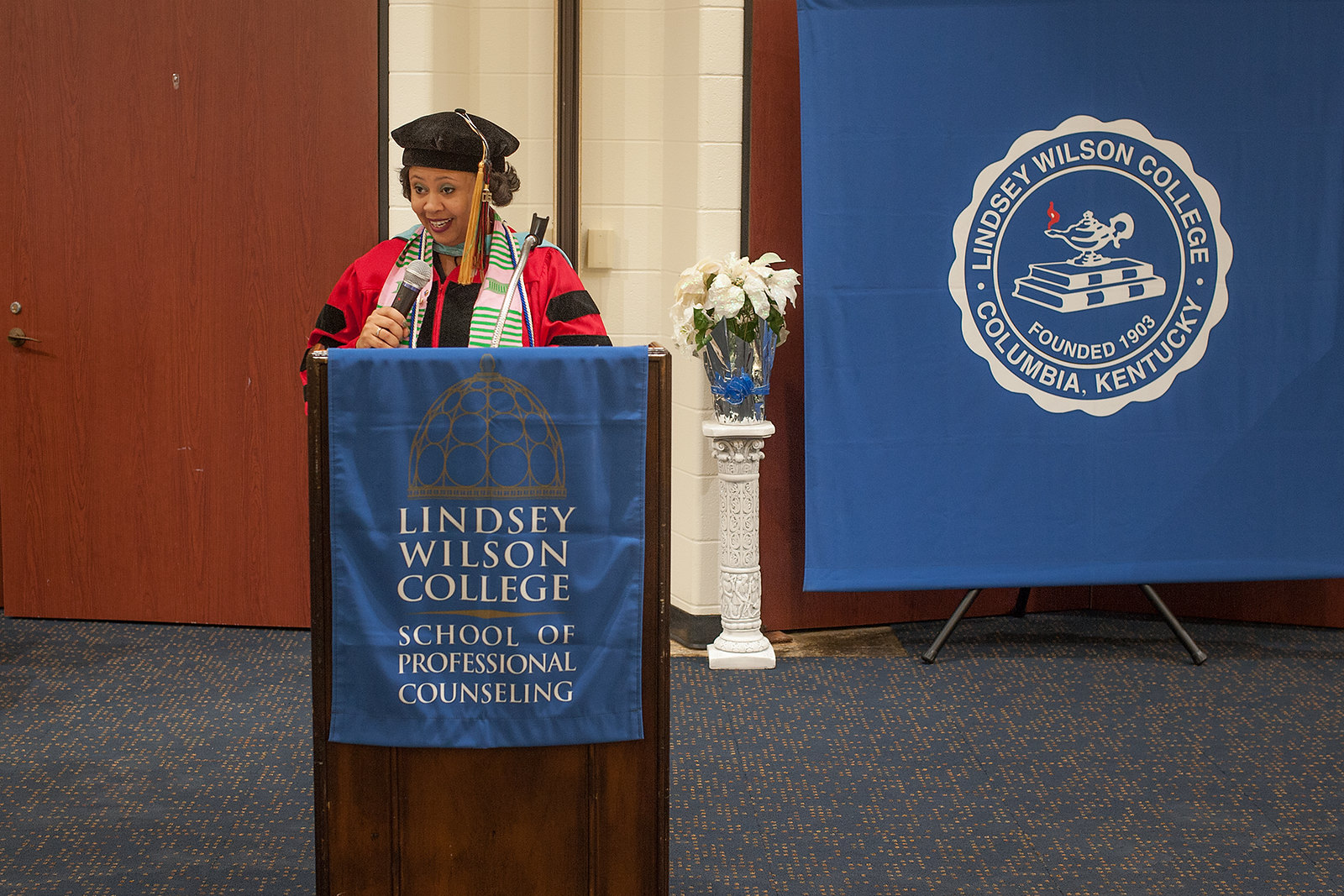The image depicts a young African-American woman standing at a wooden podium adorned with a banner reading "Lindsay Wilson College, School of Professional Counseling." She is dressed in a red graduation robe with black stripes and wears a black graduation cap with a tassel hanging to the left. The woman holds a microphone in her hand, and draped across her neck is a blue scarf that cascades down her back, along with a pink and green striped scarf hanging down her front. Behind her, a large door and brown and white walls frame the scene, while a pedestal with a vase of flowers adds a touch of elegance. The blue speckled rug on the floor completes the setting. Additionally, another banner in the background proclaims "Lindsay Wilson College, Columbia, Kentucky, founded in 1903" and features a stack of books and a genie lamp.